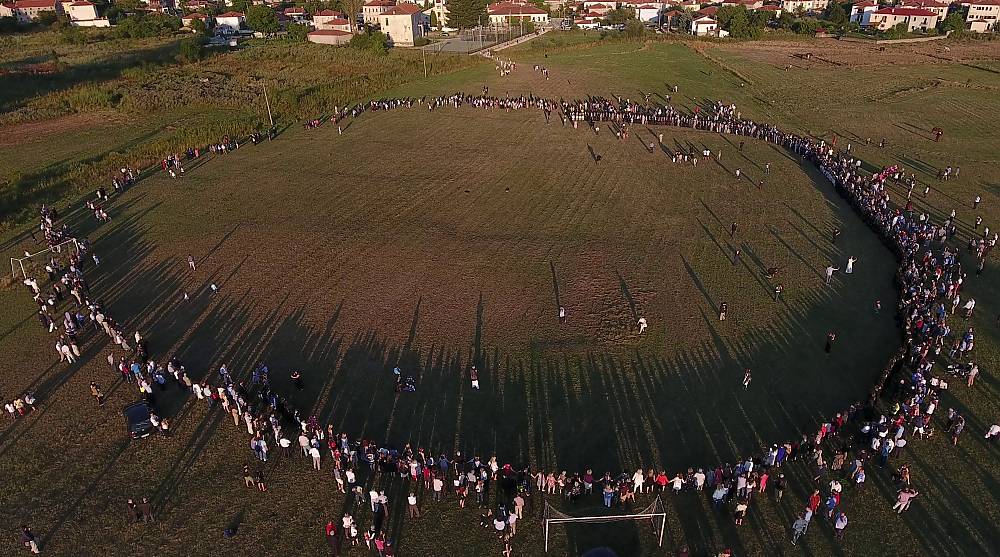The aerial photograph captures a large, grassy field in a suburban neighborhood, surrounded by tan houses with brown roofs. The central focus of the image is a massive circle of several hundred people gathered on the flat, clean ground, with the circle expanding wide enough to make the individuals appear small in the vastness of the open space. While most people form the circle, a few wander outside it or stand scattered within its bounds. Notably, the bottom section of the image reveals a soccer net, hinting at a possible sports-related gathering, though the circular formation of the crowd adds an element of intrigue. Long shadows stretching across the scene suggest that the photo was taken late in the day.